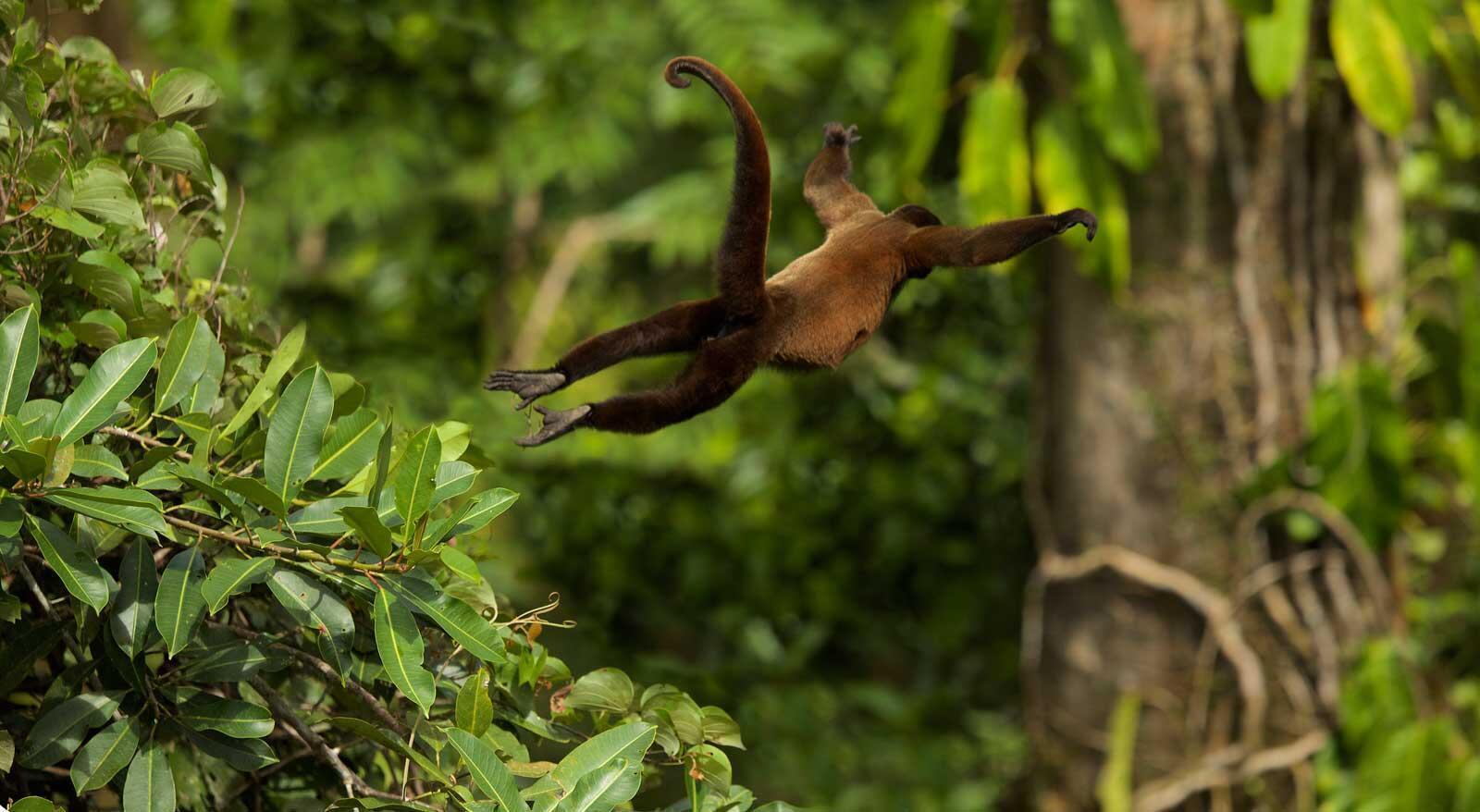In this lush, green outdoor woodland scene, a monkey, possibly a howler monkey, is captured in mid-leap. The background is filled with vibrant green leaves and dense vegetation. On the left side of the image, one can see green leaves and part of a bush, contributing to the forest's dense undergrowth. Dominating the right side is a prominent, thick brown tree trunk. This tree, although significantly large, appears distant and slightly out of focus.

The foreground features the monkey in a dynamic, airborne pose resembling a "Superman" flight. Its light brown torso contrasts with its long, dark brown legs, tail, and arms. The monkey is mid-jump, with its arms extended forward and its body angled upward, conveying a sense of motion and energy. The upward-pointing tail and stretched-out legs underscore the mid-air acrobatics. The daylight filtering through the canopy reveals patches of sunlight, enhancing the vividness of this natural spectacle. The monkey, seemingly leaping from a branch or the forest floor, is framed perfectly amidst the greenery, embodying the wild essence of its habitat.